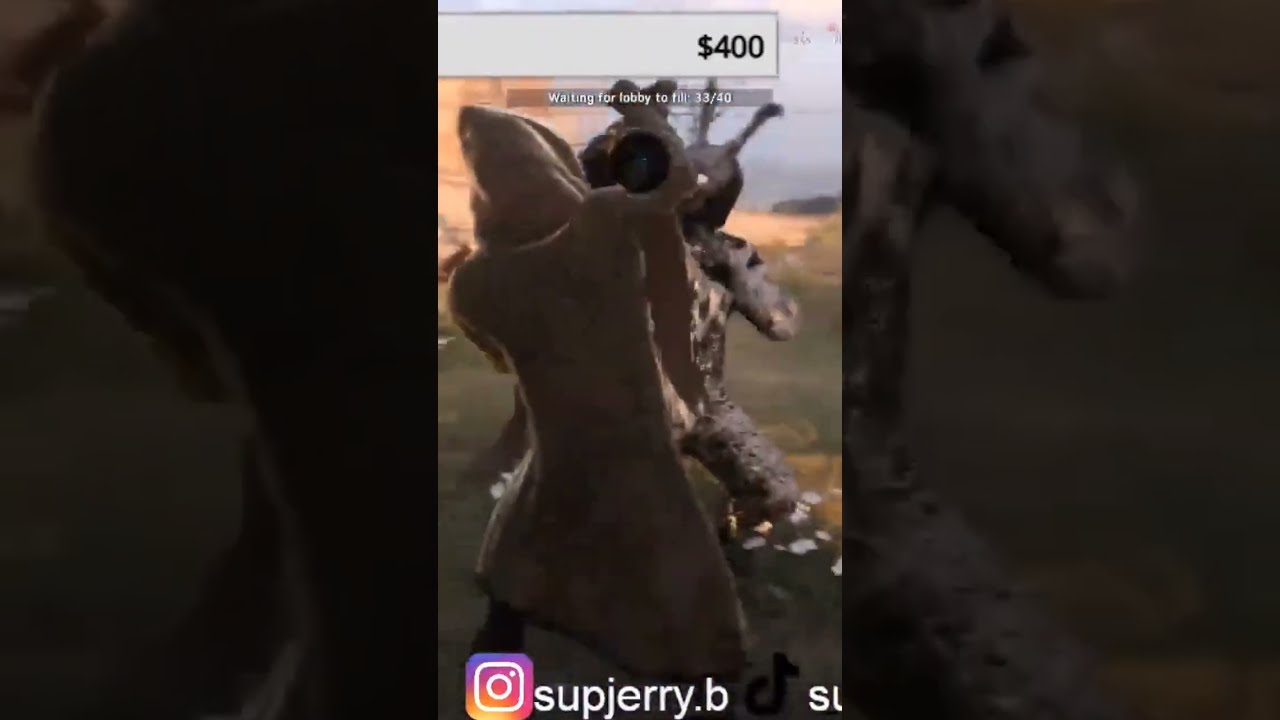The image is a screenshot from a video game, depicting two figures engaged in a battle. The scene seems slightly blurry and possibly set in a desert environment. One figure, clad in a long hooded coat (possibly brown) with their back to the camera, is facing another figure in camo attire, who has a mask with tall antenna-like extensions. Their faces are obscured, adding to the mysterious and tactical vibe. At the top of the screenshot, a white banner displays "$400.00" in slim black lettering. Just below this, text reads "waiting for lobby to fill 33/40." The bottom of the image features an Instagram camera icon followed by the handle "SUPJERRY.B" in white print. Overall, the screenshot captures a moment of intense confrontation between two heavily equipped characters in a rugged setting.